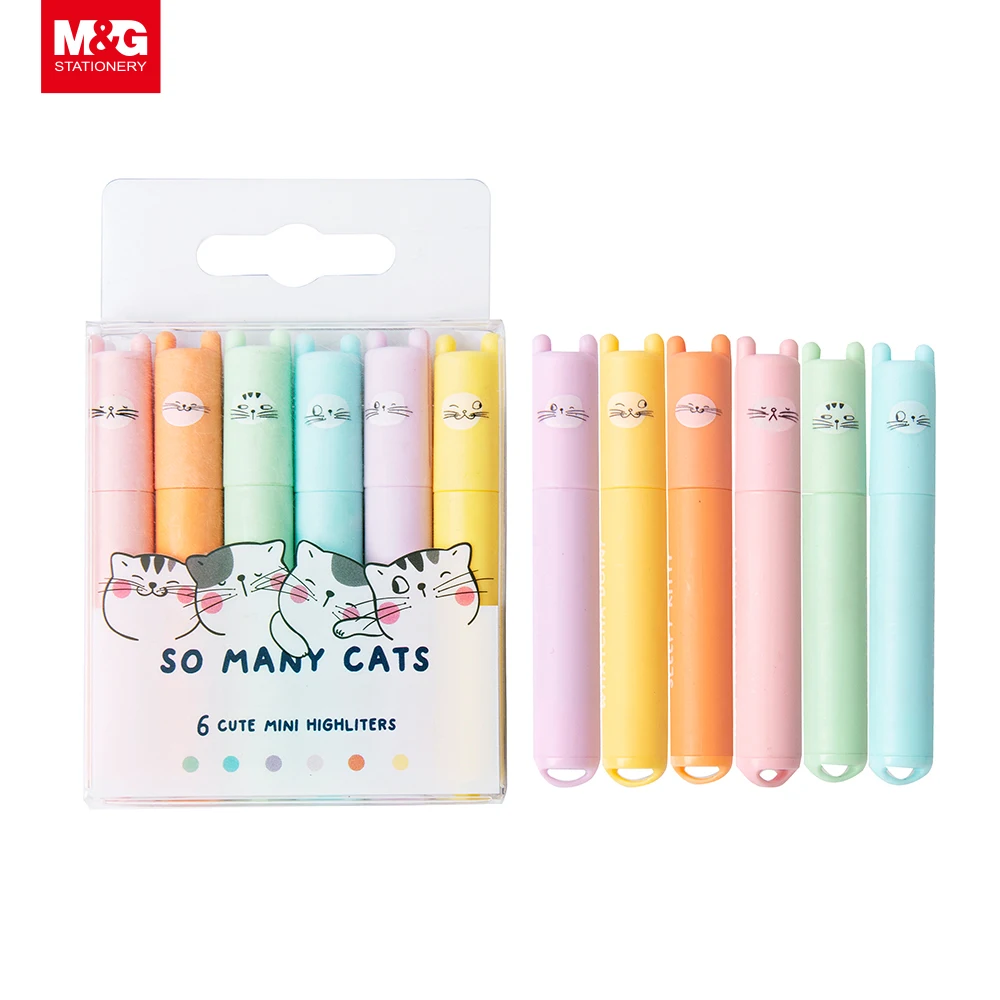In this image, set against a white background, we see a package of six cute mini highlighters from M&G Stationery, identifiable by their red logo at the top left. The package prominently features the text "So Many Cats Six Cute Mini Highlighters" in blue. The highlighters are displayed both inside and outside the transparent container. Each highlighter is pastel-colored—pink, yellow, orange, green, blue, and purple—and topped with caps designed to resemble cat ears. Each highlighter also features adorable cat faces displaying various expressions such as winking, smiling, and looking in different directions. The overall packaging and design emphasize a playful, cat-themed aesthetic, with four additional cat portraits decorating the middle of the package.